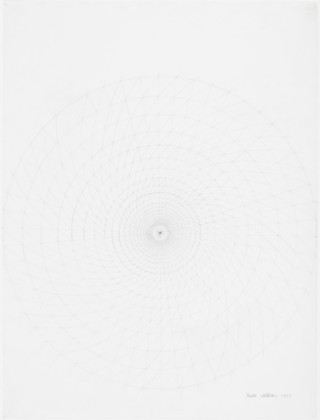This is an extremely subtle and minimalist graphic painting presented in portrait orientation. The predominant color is a very light gray, almost white or off-white. At first glance, it may appear as though the image has not fully loaded or is simply a blank canvas. However, upon closer inspection, one can discern a dark charcoal dot precisely located in the center of the painting. Surrounding this central dot is a series of meticulously drawn concentric circles that gradually fade into the background color, making them nearly imperceptible. Additionally, towards the very bottom right-hand corner, there appear to be a couple of small splotches, which might be the author's signature or another form of subtle marking. The artwork’s simplicity and uniform light gray background require careful attention to appreciate the intricate details and patterns, including the subtle crisscross or spiraling lines interwoven with the concentric circles.